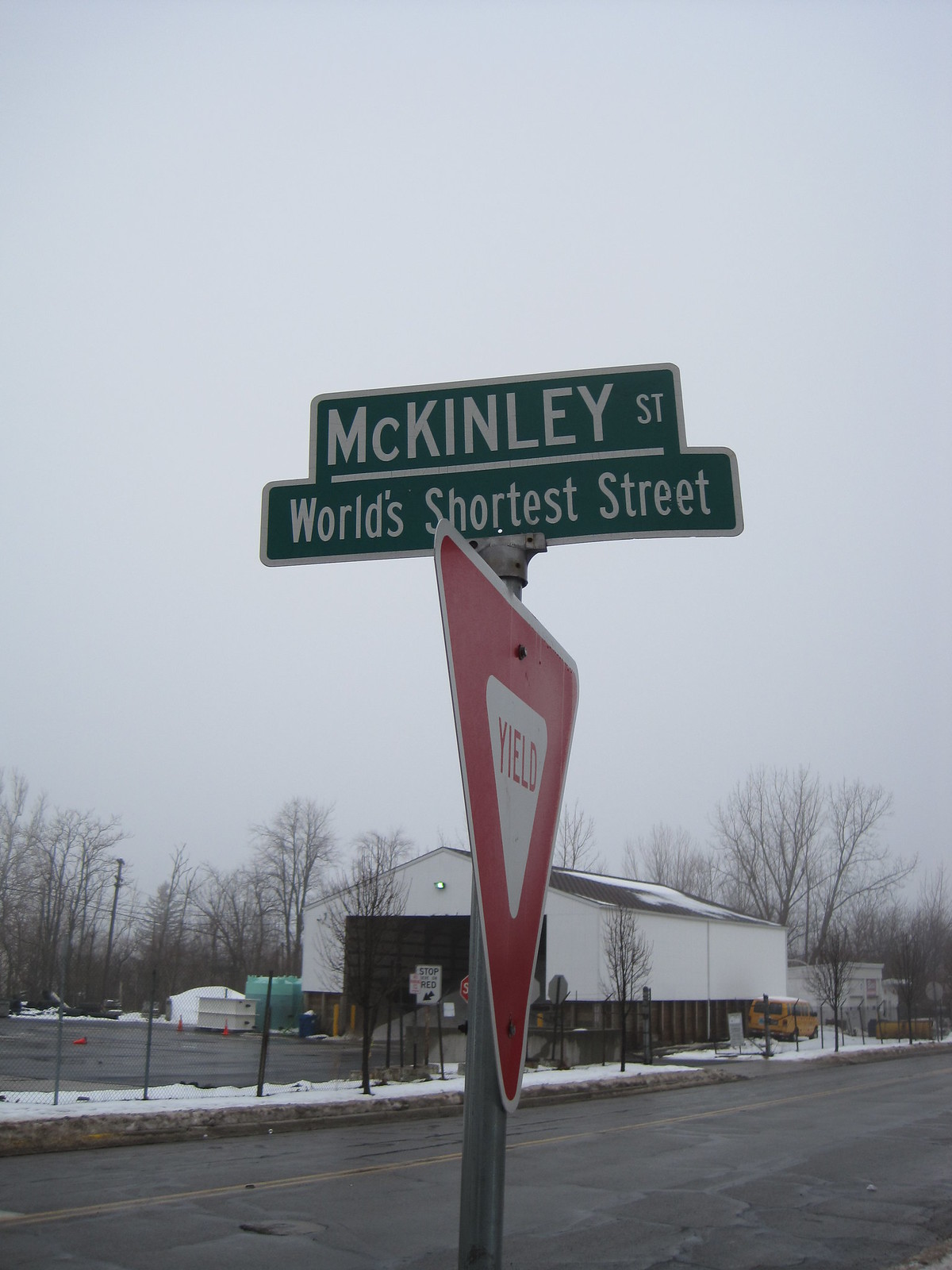In this image, we have a close-up of a green street sign that reads "McKinley Street, world's shortest street" in white lettering. Below it, a red and white yield sign is visible from the back. The surrounding environment includes a warehouse or storage building in the background, while the ground is blanketed in white snow. The street itself appears dark and wet, indicative of recent snow and slush. The skies above are dark grey, adding a somber tone to the scene, and the trees in the background are starkly bare, devoid of leaves.